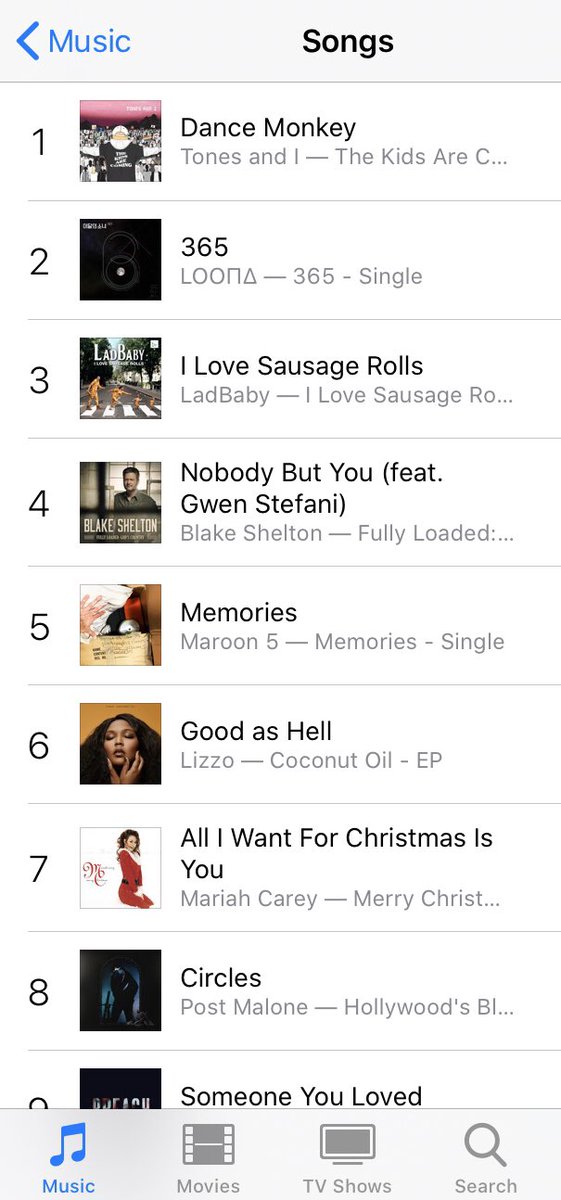The screenshot depicts an iOS device, likely an iPhone, displayed in portrait mode. The image showcases the "Music" section within the iTunes app, as indicated by the blue-highlighted music icon on the footer. Other selectable tabs include Movies, TV Shows, and Search. At the top, a left-facing arrow serves as a back button, next to which "Music" is displayed in blue text. The "Songs" category is prominently bolded in the center of the header.

The screenshot lists nine songs, with the partially visible ninth song, each accompanied by an album cover or song image on the left. Each entry is numbered and includes a subtitle for additional information. The songs listed are:

1. "Dance Monkey"
2. "365"
3. "I Love Sausage Rolls"
4. "Nobody But You" (featuring Gwen Stefani)
5. "Memories"
6. "Good As Hell"
7. "All I Want For Christmas Is You"
8. "Circles"
9. "Someone You Loved" (partially visible)

The layout is typical of a music chart or playlist, providing a clear, organized display of top music tracks.